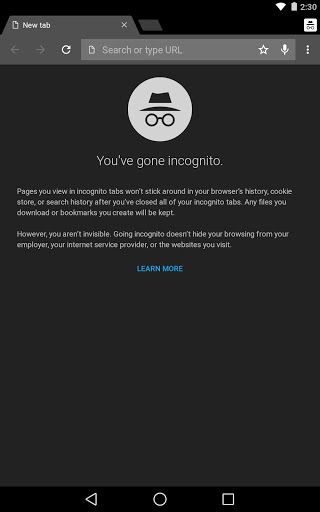A screenshot showcasing a browser window in incognito mode against a black background. At the top, the current time is displayed as 2:30, next to a search bar with a left arrow, right arrow, and a white refresh button. Other standard browser buttons are visible in gray, and there are three vertical dots for additional options. To the right of the search bar, there is a star icon and a microphone icon. Below, a circle with a hat and glasses icon indicates that the incognito mode is active, accompanied by the message: "You've gone incognito. Pages you view in incognito tabs won’t stick around in your browser’s history. Cookies, or search history will not be preserved after you’ve closed all of your incognito tabs. Any files you download or bookmarks you create will be kept. However, you are not invisible. Going incognito doesn’t hide your browsing from your employer, your Internet service provider, or the websites you visit." There is an option to "Learn more" highlighted in blue. At the bottom of the window, three icons are displayed: a triangle pointing to the left, a circle, and a square.